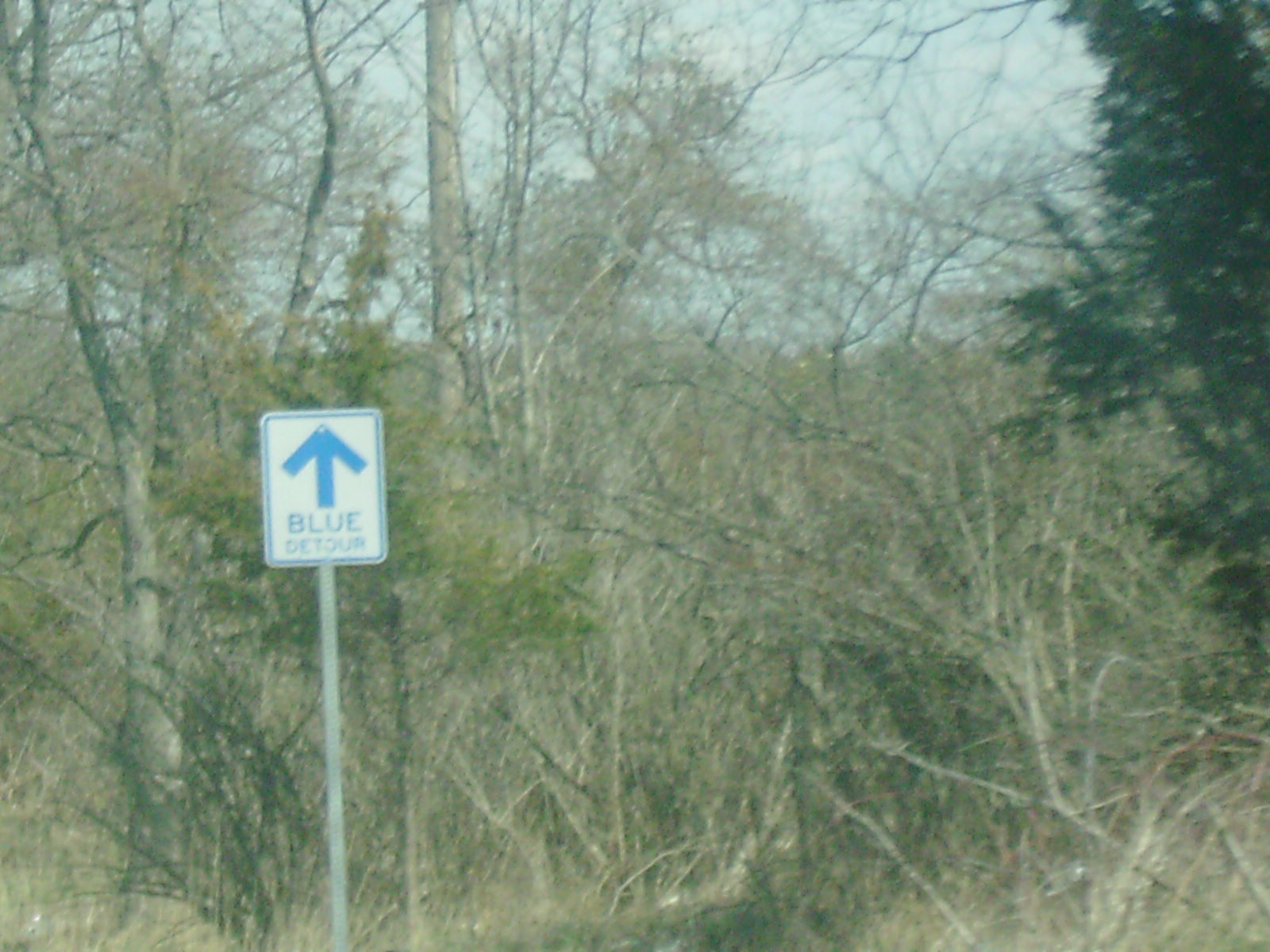The image, taken from the road, shows a forest scene with an abundance of trees, most of which are bare and brown, suggesting it is either winter or early spring. A few trees display patches of greenery, indicating the possibility of spring. Dominating the left side of the image is a long gray pole with a square sign, which features a white background outlined in blue. The sign, positioned about eight inches from the bottom of the photo, displays a thick blue arrow pointing upwards with the words "Blue Detour" written beneath it. The background of the image reveals a scattering of brown grass and tangled, unmanicured tree branches, with some trees having dark green foliage, particularly a pine tree in the upper right corner. The sky is a clear blue, visible through the web of branches, and the overall scene suggests a decent weather day. Though the picture appears slightly blurry as if zoomed in, it captures the essence of a secluded roadside area enveloped by nature’s raw, untamed growth.